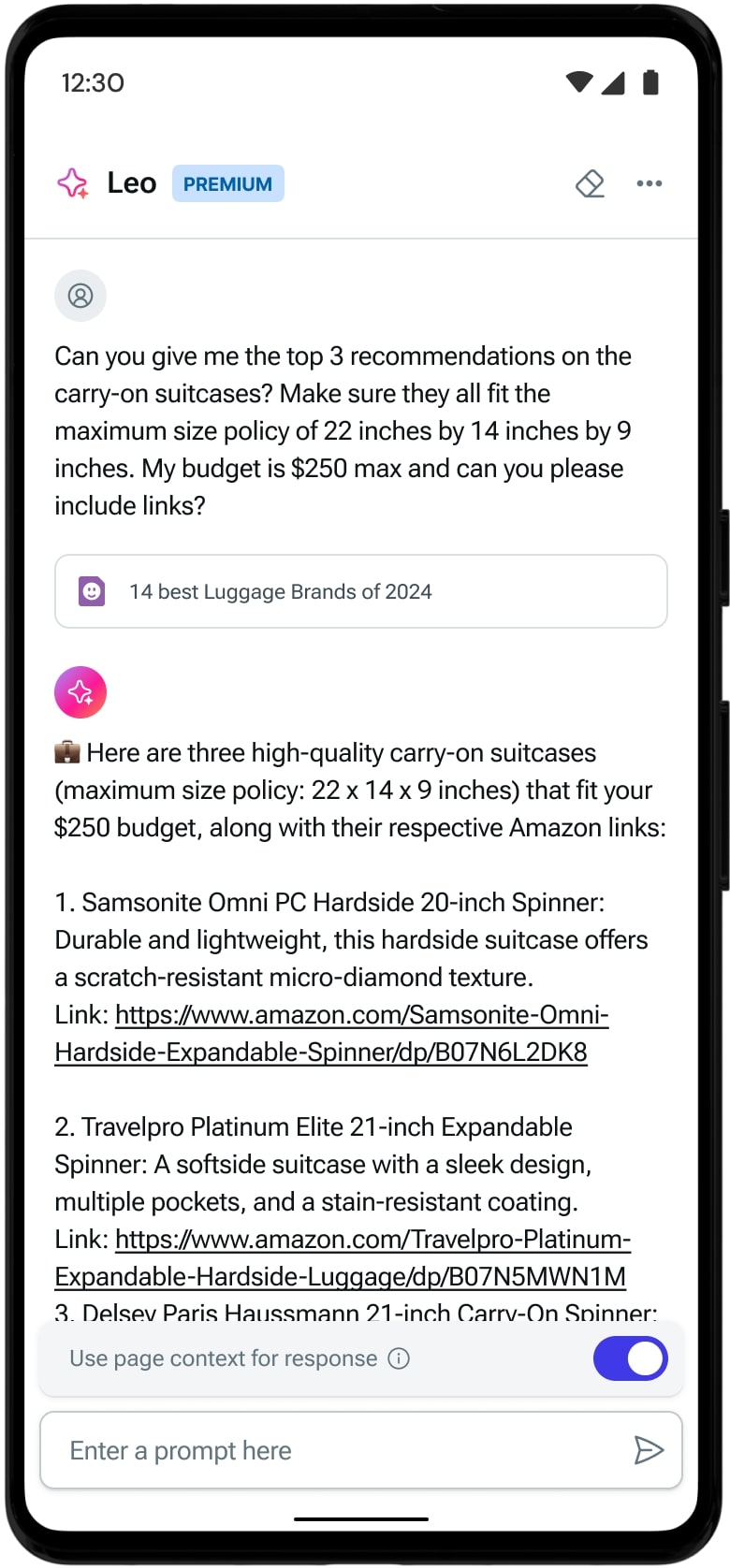This is a detailed caption for an image of a smartphone screenshot:

---

The screenshot displays a smartphone interface with a black border surrounding the screen. In the upper left corner, the time "12:30" is shown in dark text. On the upper right, several icons are visible: a diamond-shaped signal icon, a half-triangle pointing downward, and a blacked-out battery symbol. Below these icons, to the left, is a pink star with a small plus sign between its bottom and right points. Adjacent to the star, there is a black "L" followed by "EO." Next to this text is a light blue rectangular box with the words "PREMIUM" in dark blue, all capital letters.

Further down, there are two diamonds with gray borders and white interiors on a white background. A small black-gray line extends from the bottom diamond's tip toward the right, and there are three black-gray dots aligned in the middle right of this section.

Below these elements, there is a light gray circle containing a darker gray circle inside, resembling a head and shoulders icon. Adjacent to this icon, the text in dark gray letters reads: "Can you give me the top three recommendations on the carry-on suitcases?" followed by "Make sure they all fit the maximum size policy of 22 inches by 14 inches by 9 inches. My budget is $250 max. Can you please include links?"

Beneath this query, a gray rectangular box contains a smaller purple smiley face icon with white details. To the right of this, in gray text, it says, "14 Best Luggage Brands of 2024," with "L" and "B" capitalized.

Underneath is a red circle enclosing a white diamond shape with a tiny white dot between its bottom and right points. Next to it is a small, blackish, camera-like icon. The text following it reads: "Here are three high-quality carry-on suitcases (maximum size policy: 22 x 14 x 9 inches) that fit your $250 budget, along with the respective Amazon links:"

1. **Samsonite Omni PC 20-inch Spinner**: **Durable and lightweight**, this hard case suitcase offers a **scratch-resistant micro-diamond texture**. [Link: https://www.amazon.com/Samsonite-Omni-Hardside-Expandable-Spinner/dp/B07N5L2DK8]

2. **Travelpro Platinum Elite 21-inch Expandable Spinner**: A **softside suitcase** with a **sleek design**, multiple pockets, and a **stain-resistant coating**. [Link: https://www.amazon.com/Travelpro-Platinum-Expandable-Hardside-Spinner/dp/B075MWN1M]

3. **Delsey Paris Helium Aero 21-inch Carry-On Spinner** (partially cut-off but inferred from context).

At the bottom of the screenshot, there is a light gray box with the text "Use Page Context Response" in light gray letters, including a circle with an 'I' beside it. To the right of this message is a dark blue circle with a white rounded icon in its center. At the very bottom, a gray-bordered rectangular area contains the text "Entry Prompt Here" with an envelope icon pointing to the right.

There is also a thin black line running horizontally at the bottom of the smartphone screenshot.